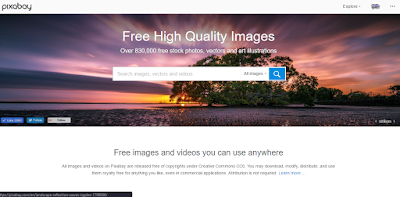The image features a promotional banner for Pixabay. In the top left corner, the text "Pixabay" is prominently displayed. Beneath it, centrally positioned, another text reads: "Free high-quality images - over 830,000 free stock photos, vectors, and art illustrations." Below this, there is a white search bar that prompts users to "Search photos, vectors, and illustrations - All images," accompanied by a blue search button.

The background showcases a picturesque landscape with a tall tree on the right side of the image. The tree, strikingly white and green, stands in contrast to the dark brown land. To the left of the tree, a radiant yellow sun illuminates the scene, highlighting a lake on the right. The sky overhead is filled with clouds tinged with shades of yellow, black, and purple hues due to the sun's influence.

At the bottom of the image, text announces: "Free images and videos you can use anywhere." This text, along with other smaller and blurrier text indicating that all images and videos are fake, adds contextual depth. A noticeable blue button at the bottom right says "Learn More." The textual elements are set against a white backdrop with black font.

Additionally, social media icons for platforms such as Facebook, Twitter, and Instagram are positioned on the right side, enhancing the interactive aspect of the image.